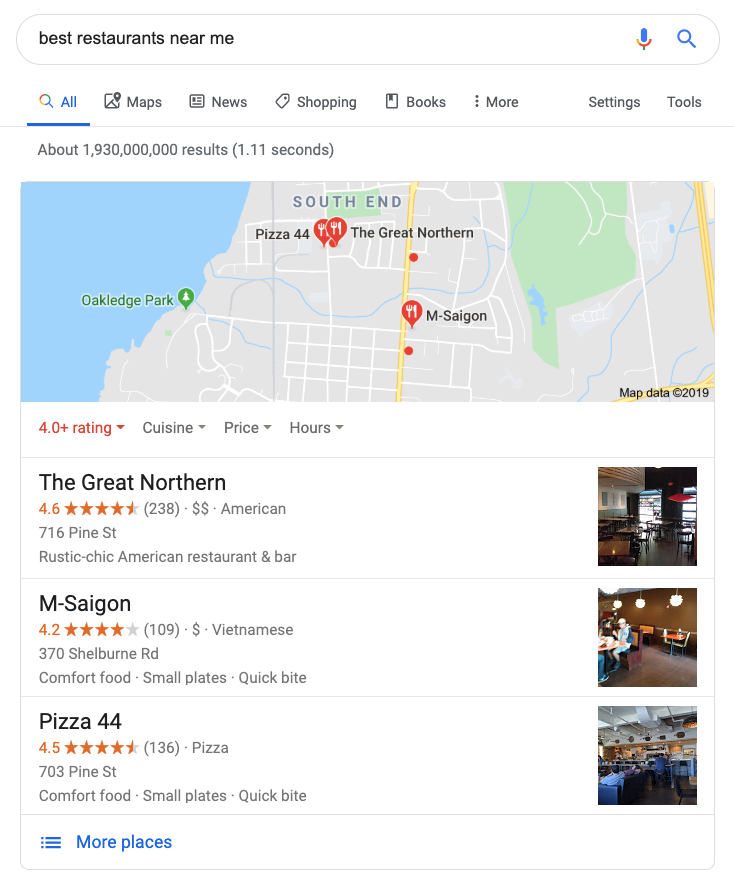The image is a screenshot of a Google search result page. At the top, there's a distinct white search bar featuring a microphone icon and a magnifying glass icon symbolizing search functionality. Inside the search bar, the query "best restaurants near me" is displayed. Beneath the search bar, there are category options outlined with a magnifying glass icon followed by tabs labeled "All," "Maps," "News," "Shopping," "Books," "More," "Settings," and "Tools." 

Below this navigation menu, the screen reveals that approximately 1,933,930,000,000 results were found in 1.11 seconds. A segment of the result includes a location map from Google Maps emphasizing the southern end of the region in question. 

Following the map, several filters such as "4.0+ ratings," "cuisine," "price," and "hours" are presented. The search results list begins with "The Great Northern," which boasts a 4.6-star rating from 238 reviews, categorized under American cuisine with a price range indicated by two dollar signs. Next is "M-Saigon," with a 4.2-star rating from 109 reviews, known for Vietnamese cuisine and depicted with a single dollar sign. 

Following is "Pizza 44," which holds a 4.5-star rating from 136 reviews and is noted for its comfort food. Each restaurant listing includes a thumbnail image showing the interior of the establishment. The restaurant names and details are in black text, while the additional information such as ratings and categories are in gray text.